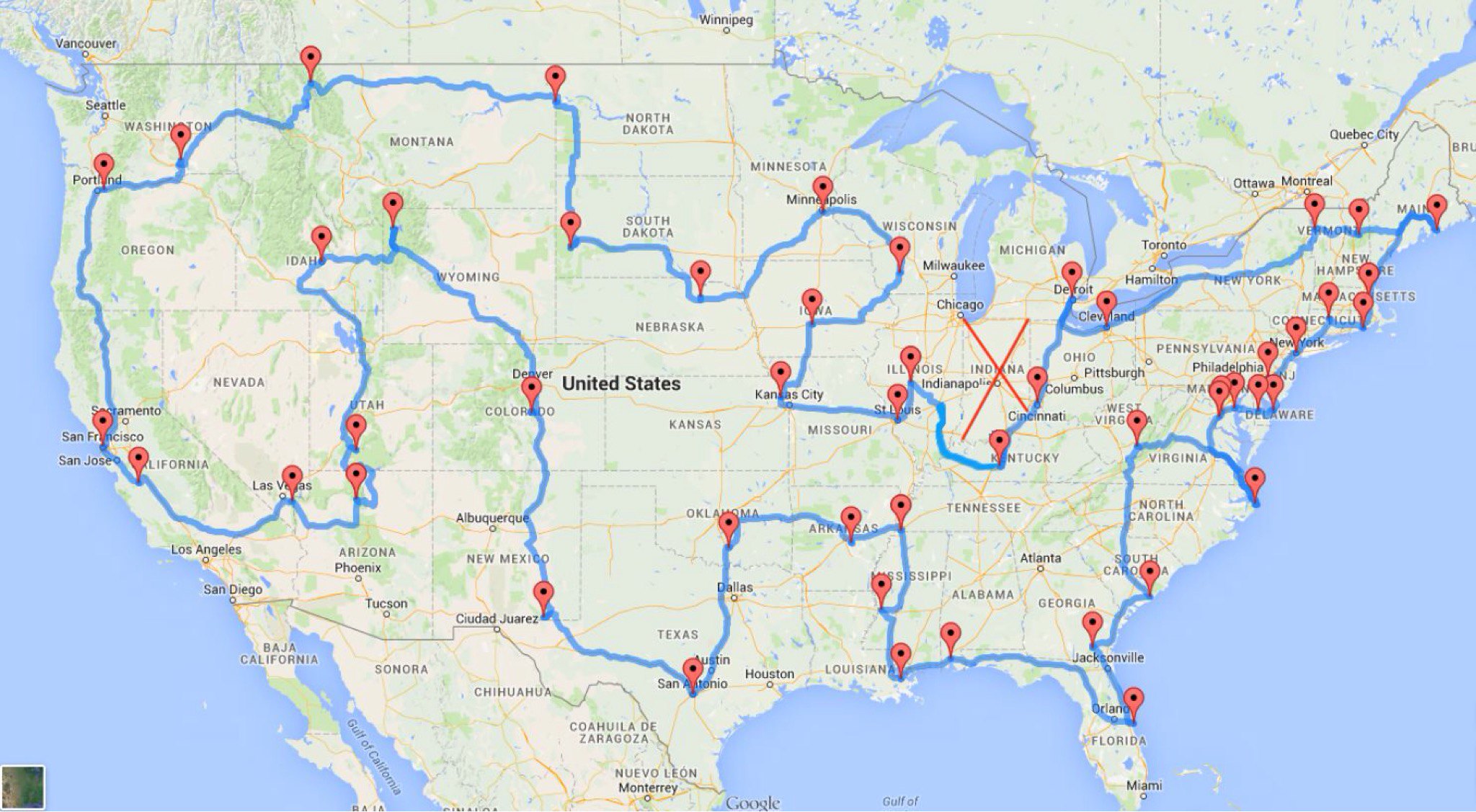This image features a detailed map of the United States. The map outlines the country's geographical layout, with the oceans depicted in blue and the mainland rendered primarily in white, interspersed with accents of green. The map prominently identifies the United States and is dotted with numerous red pointers, each highlighting major cities across the nation. In the southeast, Orlando and Jacksonville are marked in Florida. The map also highlights key locations in South Carolina, Tennessee, and Mississippi. Further west, major Texan cities such as Dallas and Houston are noted. Kansas City is pinpointed in the central region. On the west coast, significant cities such as San Jose and San Francisco in California, alongside Portland in Oregon and areas in Washington State, are similarly denoted.